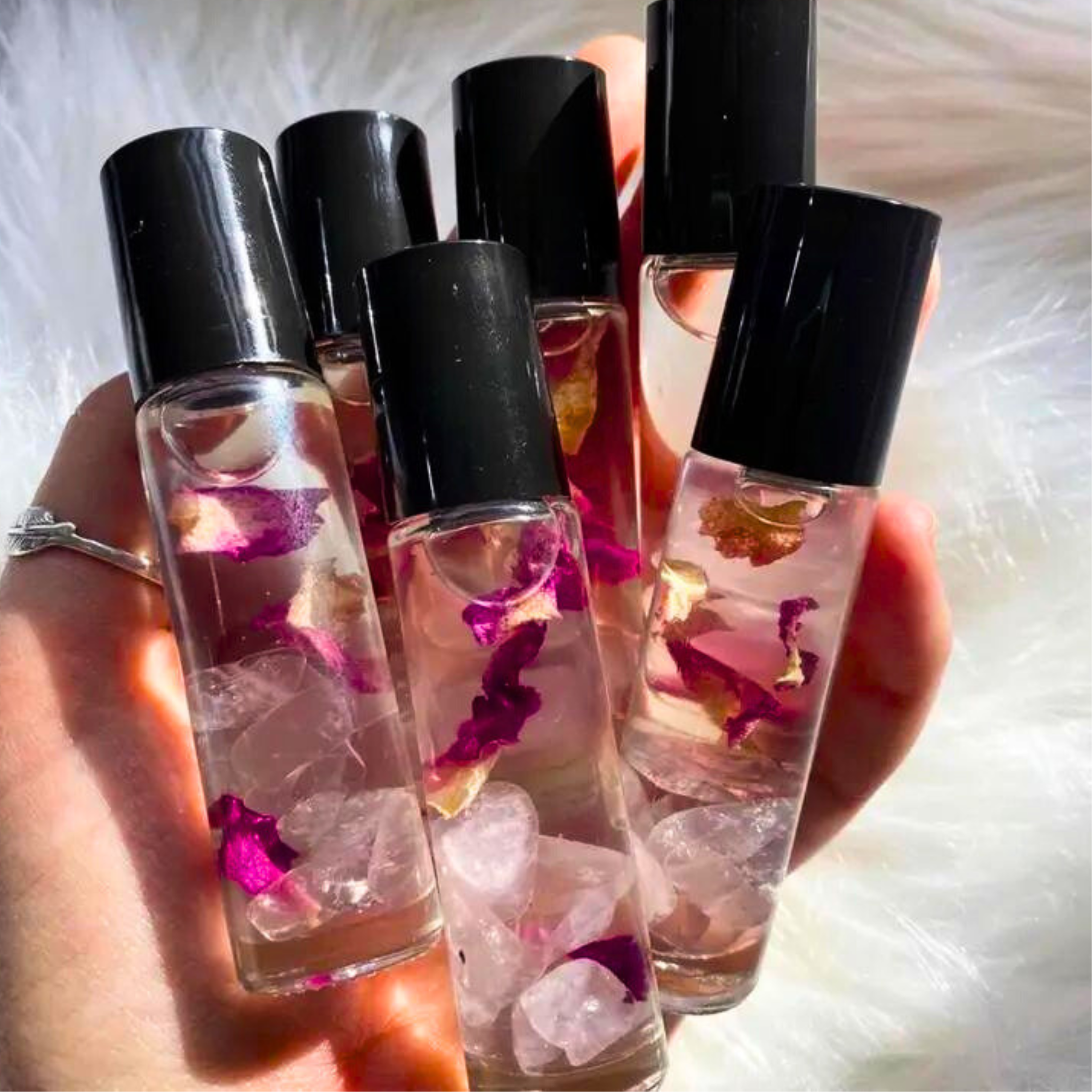In this photograph, a young woman's hand, adorned with a silver thumb ring, is displayed against a white background. Her palm is raised and open, holding six small glass vials, each with a black plastic cap. The vials are nearly filled with a clear liquid, leaving tiny air bubbles visible. Inside each vial, there are small pink flower petals and what appear to be crystal-like stones or salt pieces, adding a delicate and decorative touch to the contents. The image focuses solely on her hand and the vials, emphasizing the detailed and intriguing composition of the objects.